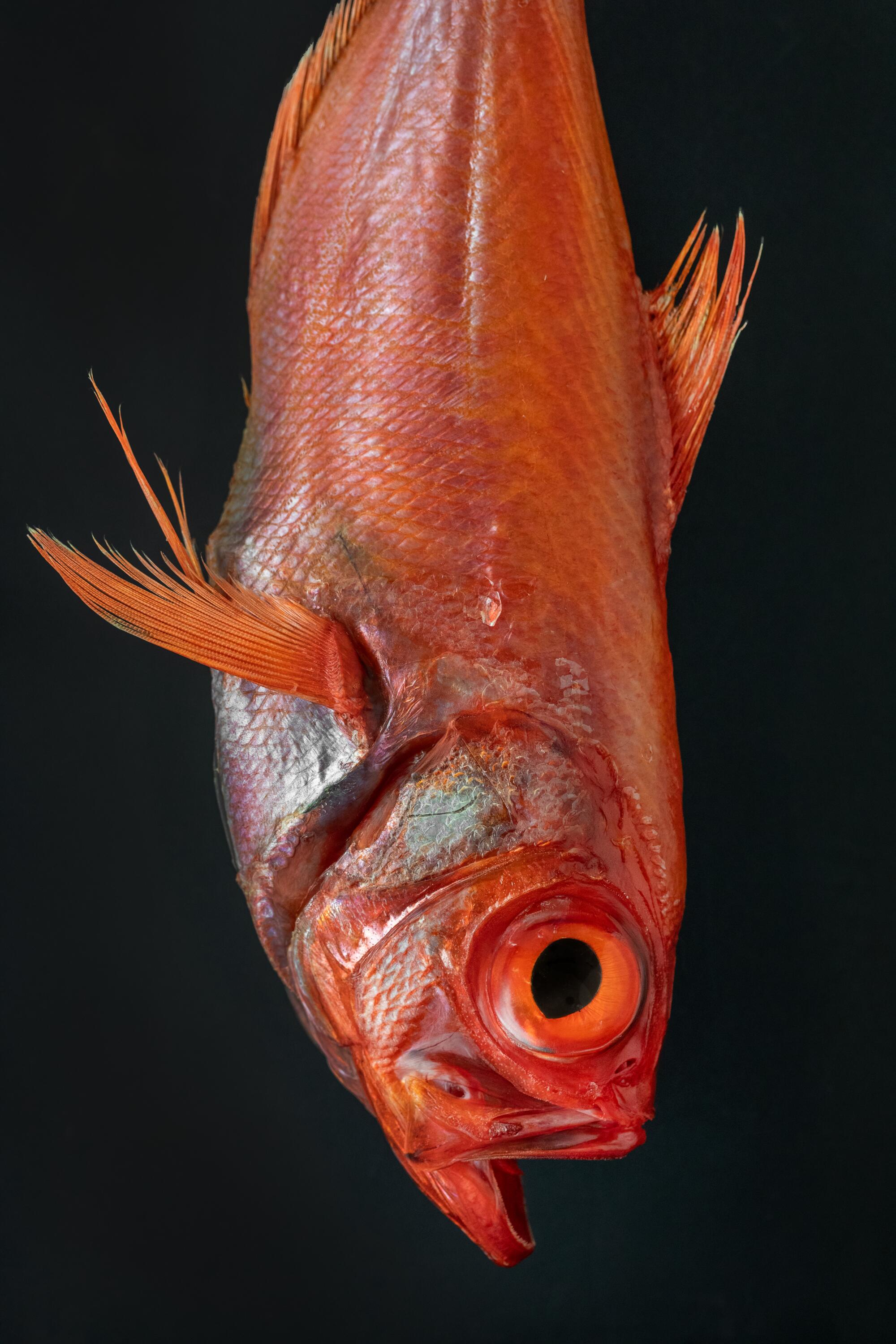The poster features a striking, close-up photograph of a deceased red fish, likely a red snapper, hanging vertically upside down against a solid black background. The fish, captured in exquisite detail, is predominantly a bright red-orange with subtle variations; its belly and regions near the gills exhibit a silvery hue. The fish's large, circular eye is an intense shade of orange with a black pupil, and its mouth is slightly open, revealing no teeth. Prominent, spiky fins extend from its side and top, while additional fins near the back lie slick against its body. The gills are clearly visible and well-defined, adding to the vivid realism of the image. The poster, rendered in a portrait orientation, powerfully contrasts the vibrant fish against the deep black backdrop, making the aquatic subject appear almost surreal in its suspended state.